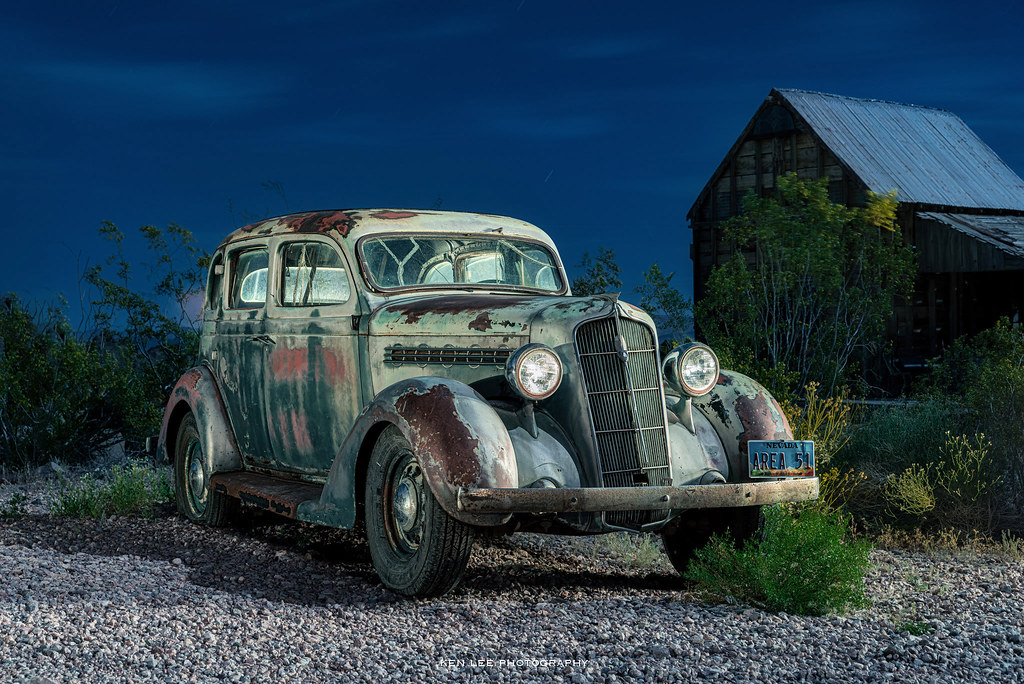This professional nighttime photograph captures a vintage 1940s-era vehicle prominently displaying a Nevada Area 51 license plate. The car, characterized by its aging patina, blends a mix of green, yellow, and white paint that is flaking away to reveal rusty undertones. Its distinctive design features include a large, vertically-oriented front grille flanked by round, globe-like headlights and a chrome exterior bumper. The car's tires show signs of neglect, with one rear tire visibly flat. The vehicle rests on a gravel surface, with sporadic green bushes and small trees scattered around.

In the background, a rustic barn with a metal roof stands against a dark blue sky, suggesting either nighttime or an impending storm. Subtle lighting enfolds the car evenly, highlighting it without the harshness of an amateur flash, implying a skilled hand behind the lens. The photograph bears the watermark "Ryan Kenley Photography," suggesting a professional touch. The image captures a faint moon glare above the car and a small green shrub in the foreground, contributing to the antique, yet timeless atmosphere of the scene.